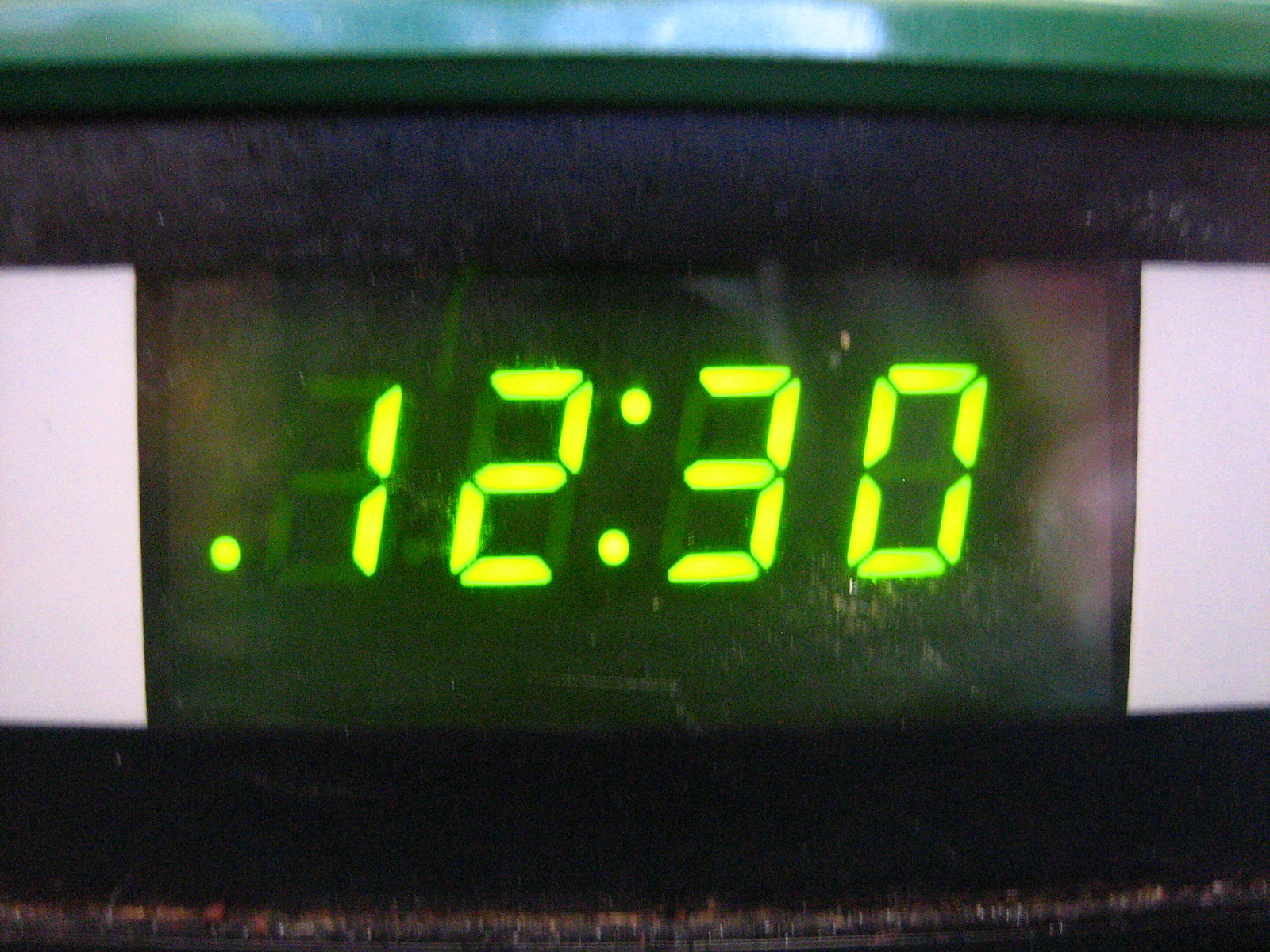The image is an extreme close-up of a digital LCD clock face against a black background. The clock displays the time "12:30" in bright yellowish-green numbers, with a layout showcasing the digits "1" and "2" on the left, followed by a colon, and then the digits "3" and "0" on the right. The clock's face is bordered by a black frame that forms a large, subtle triangle behind the numbers. This triangle spans the width of the photograph and creates a frame-like border on the top and bottom of the clock display. Adjacent to the digital screen are two blank white strips flanking either side of the clock's face. The overall image has a slightly blurry and gritty appearance, indicating that the clock is somewhat dirty and could benefit from cleaning. Additionally, a reflection is visible on the screen, and basic outlines of other possible numbers are faintly discernible, exposing the versatility of the digital display. The top edge of the photograph features a thin green strip, while the bottom edge shows some wear and tear, including a hint of yellow discoloration, which might indicate aged materials or usage wear.